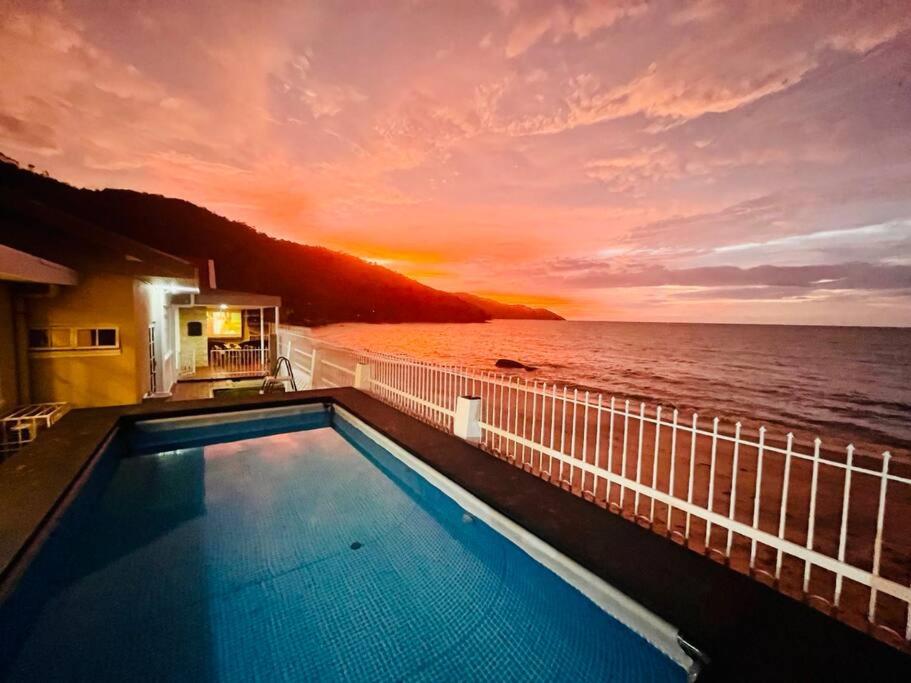The image depicts a serene coastal scene focused on a person’s boat home with multiple architectural and natural elements. In the foreground, there’s a rectangular blue pool with visible blue tile that is part of the home's outdoor area, potentially shared with a small hotel. To the left of the pool, a building with a small patio extends towards it. On the right side of the image, a white rod iron fence runs from the bottom right corner into the middle left, separating the pool area from the beach. The beach, resembling a calm cove, stretches out to a body of water colored in hues of orange and yellow, reflecting the setting sun. The horizon features large, tree-covered hills and mountains providing a picturesque backdrop. The sky is filled with patches of white clouds and is brightly lit in oranges and yellows by the setting sun behind the hill, creating a tranquil and inviting atmosphere.